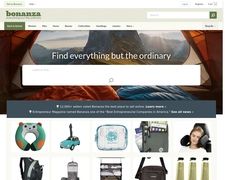The image features a collage of various elements. In the top-left corner, there's a reference to "Bonanza," although this section is somewhat unclear, appearing as a blurry, rectangular bar. Alongside the green bar to the right, numerous tabs are open on both sides of the image, creating a sense of overwhelming clutter. The center of the image showcases a majestic mountain, accompanied by text that reads, "Find everything but the ordinary." This scene is set within the context of a gray camp tent.

Below this, there's a sequence of numbers from 1 to 10, which appears to be associated with a person's pillow. Also visible in this section are a car, represented by a square shape, and a backpack placed beside other bags and various icons. The overall image is quite pixelated, making it hard to discern finer details. Additionally, there are two distinct sleeping bags — one red and one blue — along with some visible text against a light background.